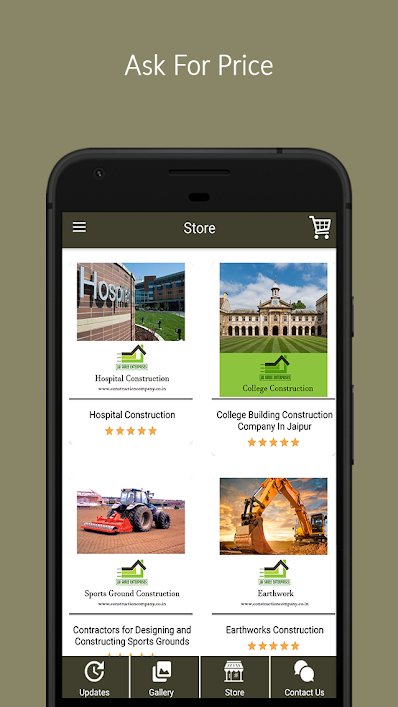A detailed caption for the image could be:

"A smartphone displays a mock-up of a construction-related website. The interface features a light gray, almost olive-colored background with white text. Prominently, the center text reads 'Ask for Price,' under which there's a photograph of an Android device showcasing the website's layout. The phone's buttons and outline are visible, indicating it's a real photograph with the screen insert added digitally. At the top of the screen, a navigation bar includes a cart icon, a hamburger menu, and the word 'Store.'

Further down, the website offers four main service options. The first option, outlined with a green house logo appearing to move laterally, is 'Hospital Construction,' featuring an exterior image of a hospital. The second highlighted option, 'College Construction,' portrays a picturesque university with a lush, green courtyard. The third option, 'Sports Ground Construction,' shows a tractor on a large, flat dirt area, indicative of initial construction stages. The final option, 'Earthwork,' displays a backhoe amid expansive dug-up dirt.

Beneath these options, the website offers detailed descriptions such as 'Contractors for Designing and Constructing Sporting Goods,' and 'Hospital Construction: Hospital Building and Construction Accompanied by JPER.' Each service is rated five stars. At the bottom, navigation links to 'Earth Updates,' 'Gallery,' 'Store,' and 'Contact Us' are available."